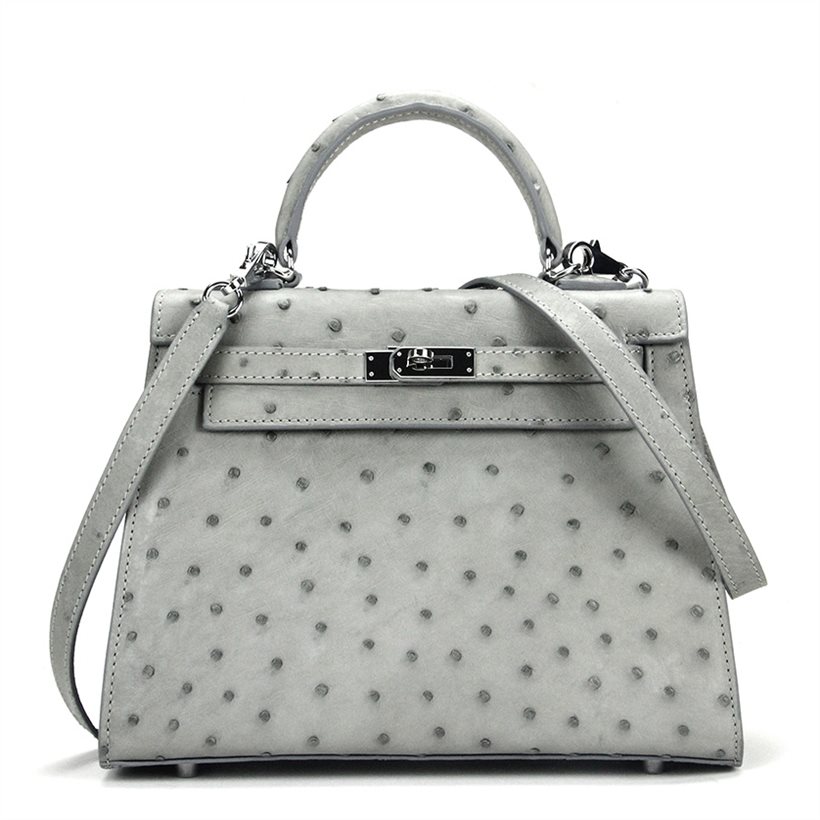The image depicts a well-crafted, designer-like purse that appears to be made from ostrich leather, characterized by its light gray color with distinctive black spots. The purse is set against a plain white background, possibly suggesting a black and white image tonally consistent throughout. It features a small, round handle at the top, complemented by a long, thin strap that seems to be tucked in or possibly removable. The hardware, including a prominent front clasp, is silver with a shiny appearance. The bag has a structured shape that narrows at the top with a wider base resembling a gusset, and white stitching adds to its detailed craftsmanship. Notably, the bottom of the bag has small legs, giving it a standing posture. Despite its resemblance to high-end designs, there is no visible label or designer name on the purse. It might be computer-generated, enhancing its sleek, modern aesthetic.